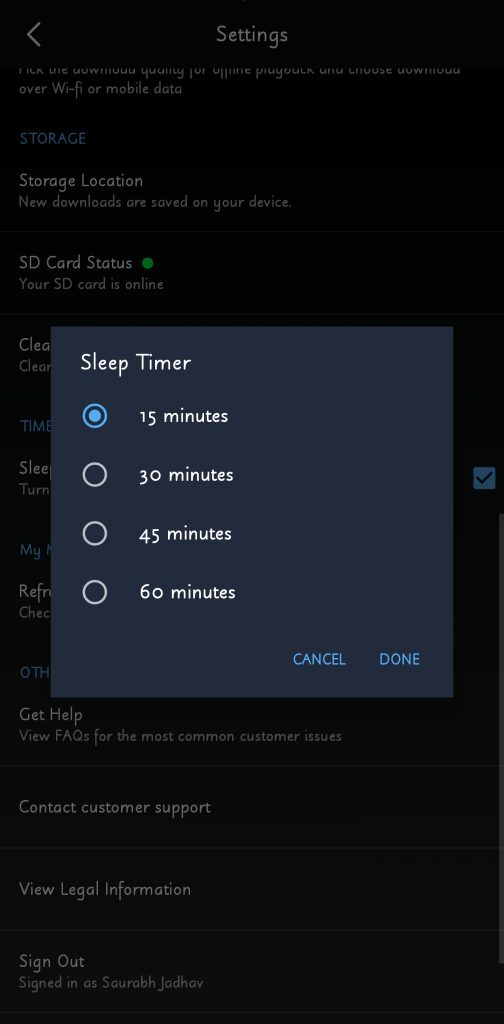Screenshot of a Sleep Timer Settings Screen on a Mobile Device:

The image showcases a black-themed settings screen on a mobile device. At the top, the word "Settings" is prominently displayed to denote the section being viewed. Below this title, a list of options is presented in white text, including "Storage Settings," "Get Help," "Contact Customer Support," "View Legal Information," and "Sign Out." 

Currently, the "Sleep Timer" option has been selected, opening a detailed sub-menu. A large blue window dominates the center of the screen, offering four duration choices for the sleep timer: 15 minutes, 30 minutes, 45 minutes, and 60 minutes. The selection of 15 minutes is highlighted by a blue circle, indicating it has been chosen by the user.

At the bottom of this blue window are two actionable buttons: "Done" and "Cancel," both colored in blue. Clicking the "Done" button will confirm and set the sleep timer to the selected 15 minutes, while the "Cancel" button will discard the current selection, allowing the user to make a different choice if desired. 

The user interface is clear and user-friendly, making it easy to set a sleep timer on this mobile device.